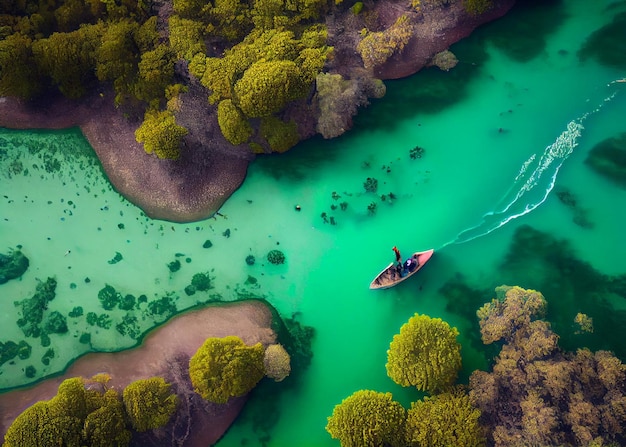This aerial photograph, likely captured by a drone, showcases a top-down view of a serene natural waterway that resembles a series of green-hued canals or lagoons. Dominating the scene is a river that courses from the upper right towards the lower left, splitting around a small sandy island. The island itself is dotted with vegetation, featuring light green to almost brownish trees with fluffy leaves. The water, which has the clear appearance reminiscent of scenes from the "Avatar" movies, is mostly still and calm, painted in an emerald green hue. One person is visible in a long, canoe-shaped boat that seems to have a motor, creating a white wake behind it in stark contrast to the tranquil water. The person appears to be navigating towards the island inlet. Surrounding the canals, additional areas of land are covered in similar verdant vegetation, occasionally extending into the water. The intricate interplay of emerald waters and lush trees captures a picturesque and dynamic landscape.